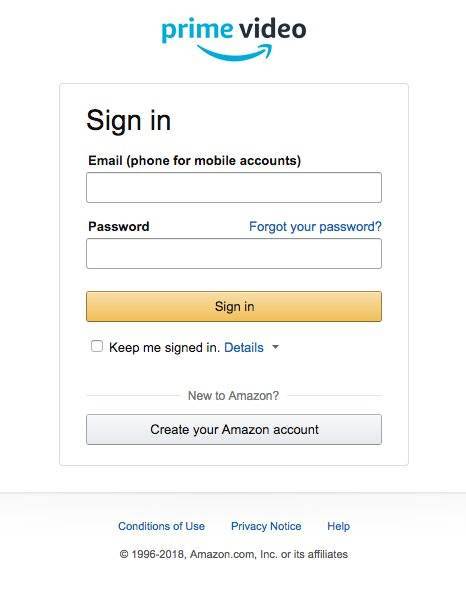The screenshot captures a login screen for the Prime Video app on a mobile device. The top of the screen, which typically displays information such as time, signal strength, and battery life, is missing. Centered at the top is the Prime Video logo, featuring "Prime" written in aqua blue and "Video" in bold black. The logo includes the distinctive swooping arrow motif in the same aqua blue color.

Below the logo is a vertically oriented sign-in form. At the top of this form, the word "Sign-In" is prominently displayed in the largest black font. Beneath "Sign-In," the text "Email (phone for mobile accounts)" is also in black, above an empty input box for email or phone entry.

Further down, "Password" is written in black, with "Forgot your password?" in clickable blue text to the right of it. There is an empty input box below for entering the password. 

The sign-in button is a light gold color with black lettering and is positioned below the password input. The option to "Keep me signed in" is unchecked, with a link to details in blue text nearby. 

At the bottom, new users are prompted with "New to Amazon?" followed by a gray button with black text that says "Create your Amazon account." The footer of the form includes links to "Conditions of Use" and "Privacy Notice," and displays the years "1996-2018" along with "amazon.com."